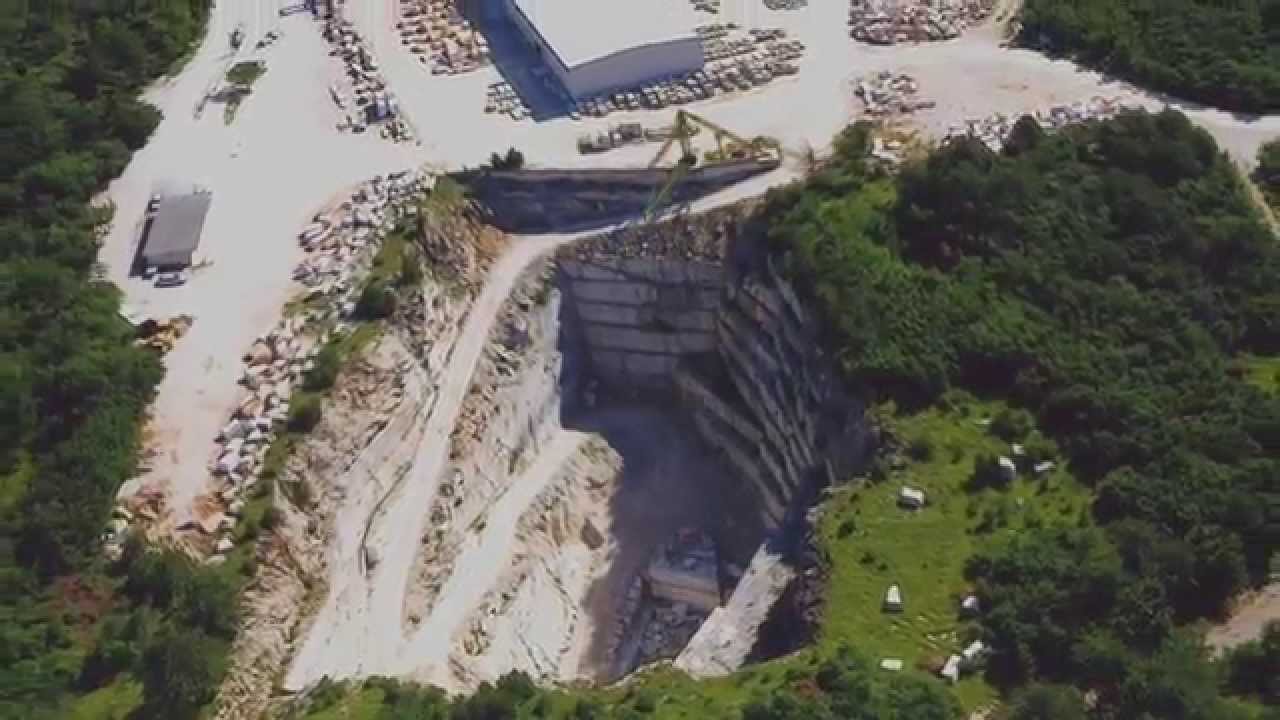This image captures a muted, aerial view of what appears to be a mining site set within a mixed landscape of forest and rocky terrain. The main focus is a significant, multi-layered excavation encircled by contrasting elements of nature and industry. The top left of the picture showcases a patch of green trees, while the middle top reveals a sandy or dirt area dotted with rocks and possibly a building, suggesting some sort of operational structure. This sandy expanse gives way to a rocky landscape, leading down into further green vegetation and eventually into a pasture at the cliff's base, where tiny white objects, presumably houses or rocks, speckle the land. There might be a winding switchback road descending into the excavation site, although the image’s poor focus and lighting make fine details difficult to discern. The photo highlights the stark juxtaposition between the greenery of the forested areas and the stark white and rocky tones of the mining site.